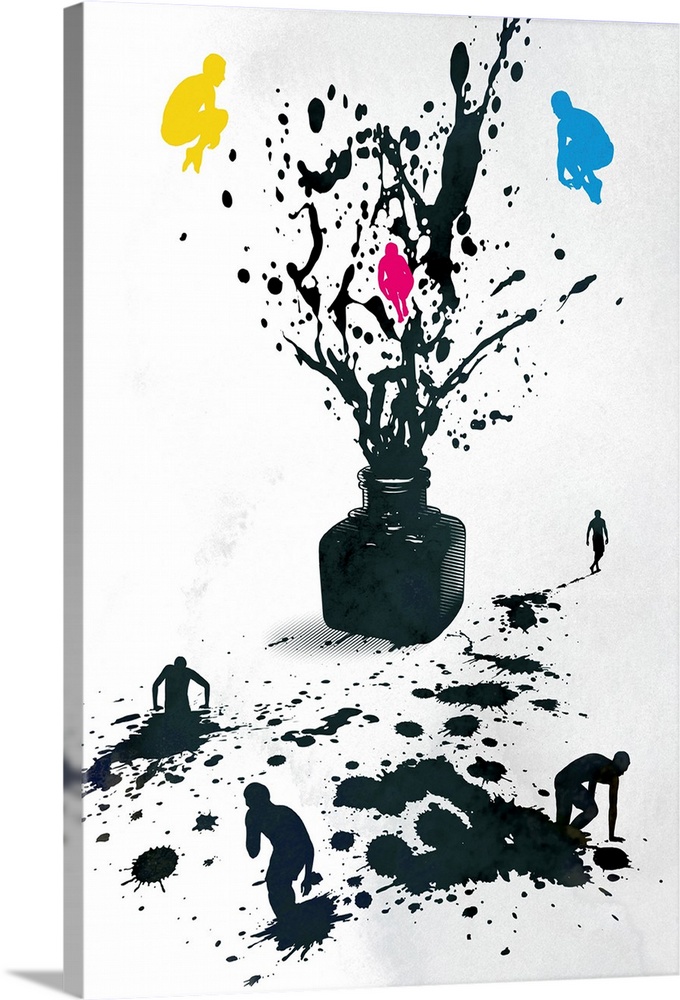This painting on a plain white canvas features a striking scene centered around a small black glass ink bottle, which appears to be explosively shooting black ink in all directions. The eruption of ink creates dramatic splotches that extend both upward and downward from the jar. Above the ink bottle, amidst the explosion, are three vividly colored silhouettes of human figures in diving poses: a yellow figure on the left, a pink figure in the center, and a light blue figure on the right, as if they have just been launched from the ink explosion. Below the bottle, the spilled ink forms a pool from which four black human-like silhouettes are emerging in various stages. One silhouette is half-submerged, another has only one foot still in the ink, a third figure is almost fully out, leaving footprints behind, and the fourth is walking away in the distance. The artwork combines the chaotic energy of the ink explosion with the detailed portrayal of human silhouettes interacting with the ink, creating a vivid and dynamic composition.